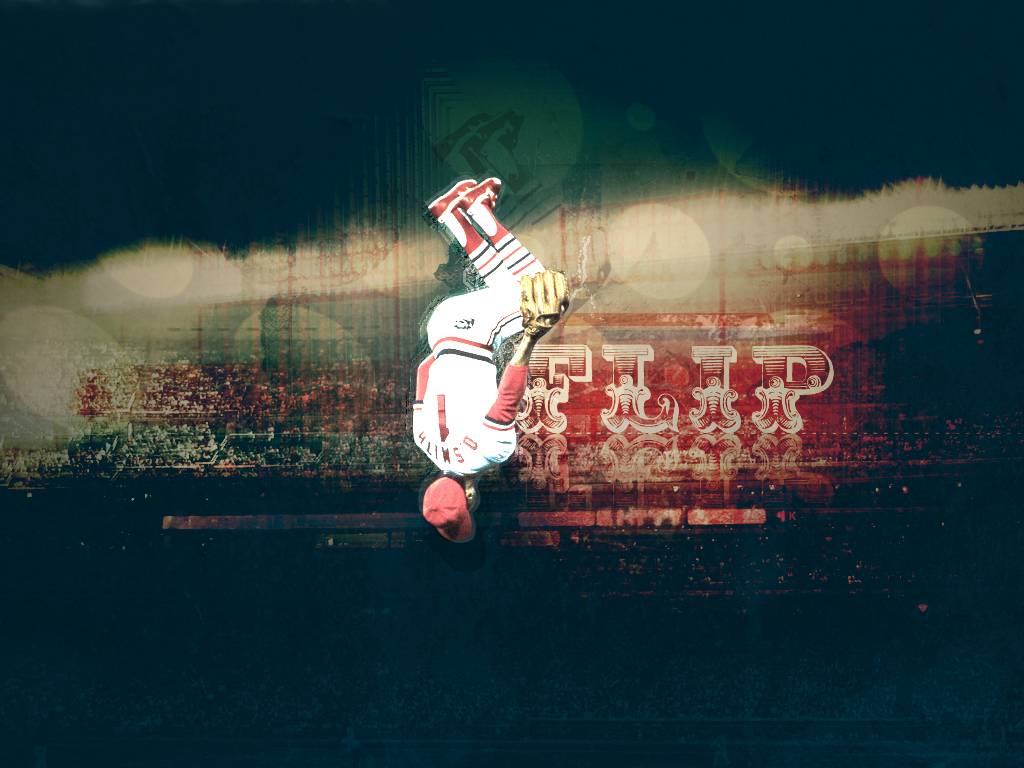The image is an artistic and abstract depiction of an upside-down baseball player, seemingly captured in mid-jump. The player wears a white uniform with red accents, including red sleeves, socks, shoes, and cap. His jersey displays the number one and a somewhat unclear name, possibly "O. Smil" or "D. Smith". The glove on one hand suggests he might be a pitcher or catcher. The background presents a high-contrast, vibrant and chaotic graphic art style, featuring a mix of city silhouettes and abstract forms in shades of green, gray, and black, interspersed with white specks. "Flip" is prominently written in a unique, ornate white font on the right side of the image, hinting at the player's dynamic action. The scene hints at a crowd in a stadium, partially visible through an overlay of shapes, giving the image an overall energetic and surreal atmosphere.